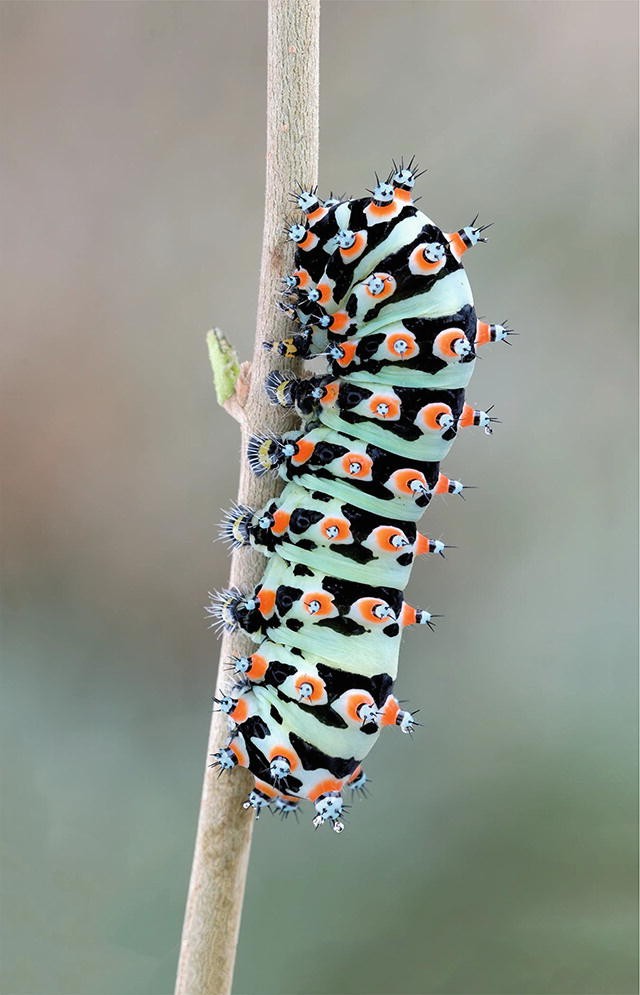In a mesmerizing macro photograph, a vividly multicolored caterpillar clings to a slender, leafless sapling. The sapling, only partially visible, emerges from the ground and fades into the blurred background, emphasizing the peculiar beauty of the caterpillar. The caterpillar itself is plump and vibrant, adorned with a pattern of blotchy black stripes over a light green, almost mint-colored body. Its skin is dotted with pimple-like protrusions, each crowned with menacing black spikes. These protrusions are mostly whitish-green, but a subtle orange tint circles their bases, adding an extra layer of complexity to its appearance. Its tiny feet, also bearing larger blackish pimples with more spikes, resemble miniature mops with white spike extensions, contributing to its oddly intimidating charm. The photograph, taken on a softly diffused bright day, captures the caterpillar and sapling in sharp detail while rendering the background an indistinct blur, creating an otherworldly yet natural scene likely fit for a nature magazine or documentary.